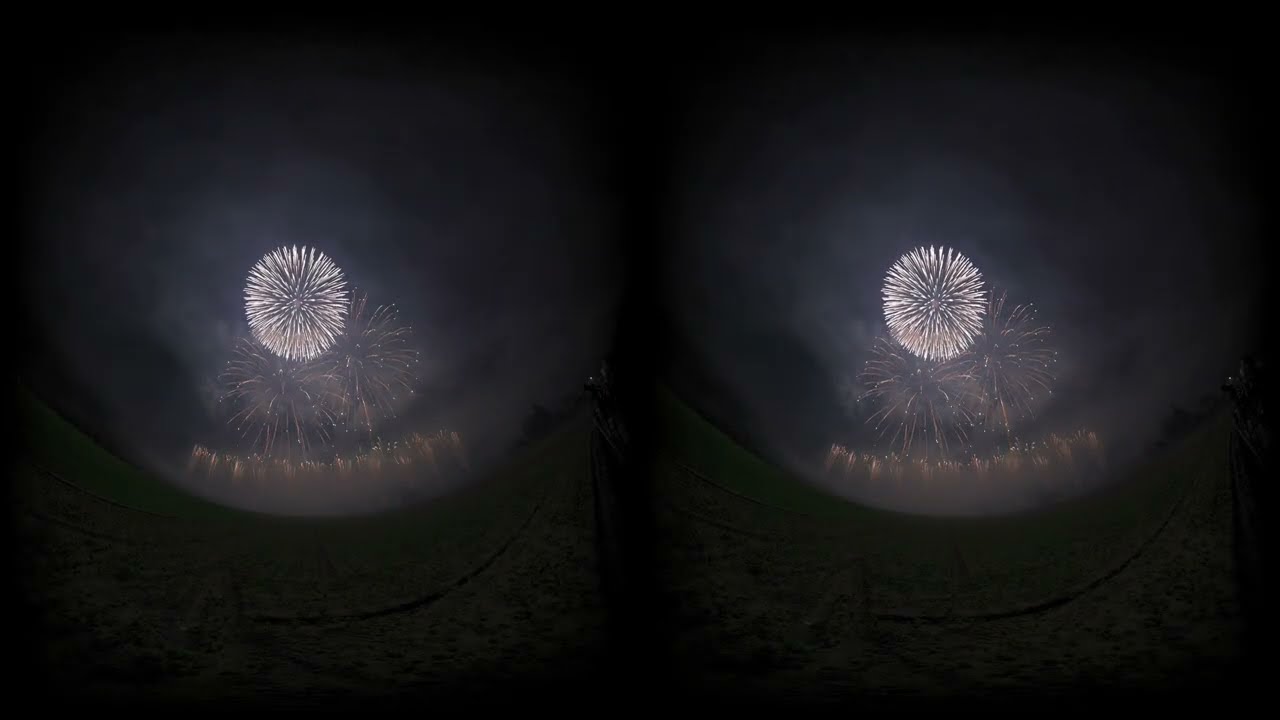The image portrays a dramatic nighttime firework display set against a pitch-black sky, possibly captured during a 4th of July celebration. Central to the scene are two prominent, white firework explosions that resemble dandelions, creating a symmetrical pattern that gives the impression of mirrored images. Beneath these larger bursts, several smaller fireworks scatter in white, adding layers to the visual depth. Despite a hint of smokiness around the explosions, the intricate design remains clear, showcasing a systematic and very pretty arrangement. At the lower part of the image, a line of differently colored amber streaks of fireworks adds to the overall spectacle. The scene also features a flat, green grass field extending towards a distant waterway, contributing to the scenic backdrop. The composition suggests a meticulous and artistic approach to the firework arrangement, possibly enhanced by an optical illusion akin to viewing through VR lenses, which bends the image slightly at the sides.